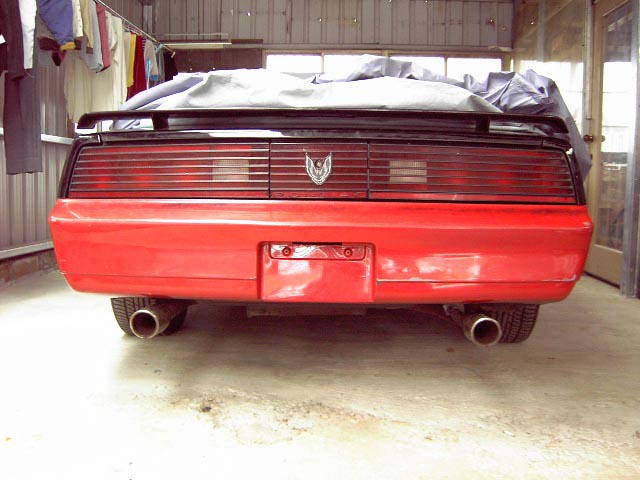The photograph captures the back end of a vintage red Firebird parked inside a brightly lit garage. The garage appears to be made of vertical metal panels painted gray. The photo, taken from the ground looking upward, shows a red rear bumper and a black spoiler, suggesting a potential two-tone paint job. Draped over the vehicle is a gray car cover, pulled back to reveal the car's distinctive features, including twin mufflers, a single long taillight divided into three sections, and a bird logo in the center. On the left side of the garage, articles of clothing hang from a rack. To the right, there is a glass wall with a door leading to another room. Bright natural lighting floods the space, enhancing the clarity and detail of the scene.